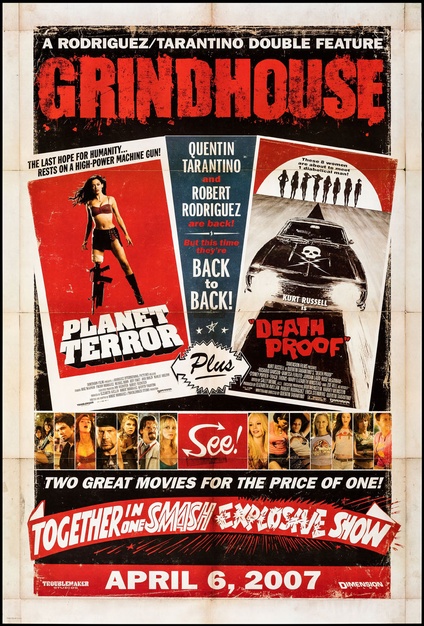This is a highly detailed movie poster advertising a Rodriguez-Tarantino double feature titled "Grindhouse," which features two films: "Planet Terror" and "Death Proof." The poster is from April 6, 2007, and promotes the event with the tagline, "Two great movies for the price of one." Dominating the center are two separate movie images. On the left side, a striking image depicts a woman with long black hair, wearing a red bikini top and dark red shorts, whose left leg is a black machine gun, representing "Planet Terror." On the right side, a black car with bright headlights and a skull emblem takes center stage, with silhouettes of women standing behind it, symbolizing "Death Proof." At the top of the poster, the text reads, "A Rodriguez/Tarantino Double Feature: Grindhouse," underscoring the collaborative nature of these back-to-back films. The poster emphasizes the unique opportunity to see both films together in one explosive showing.